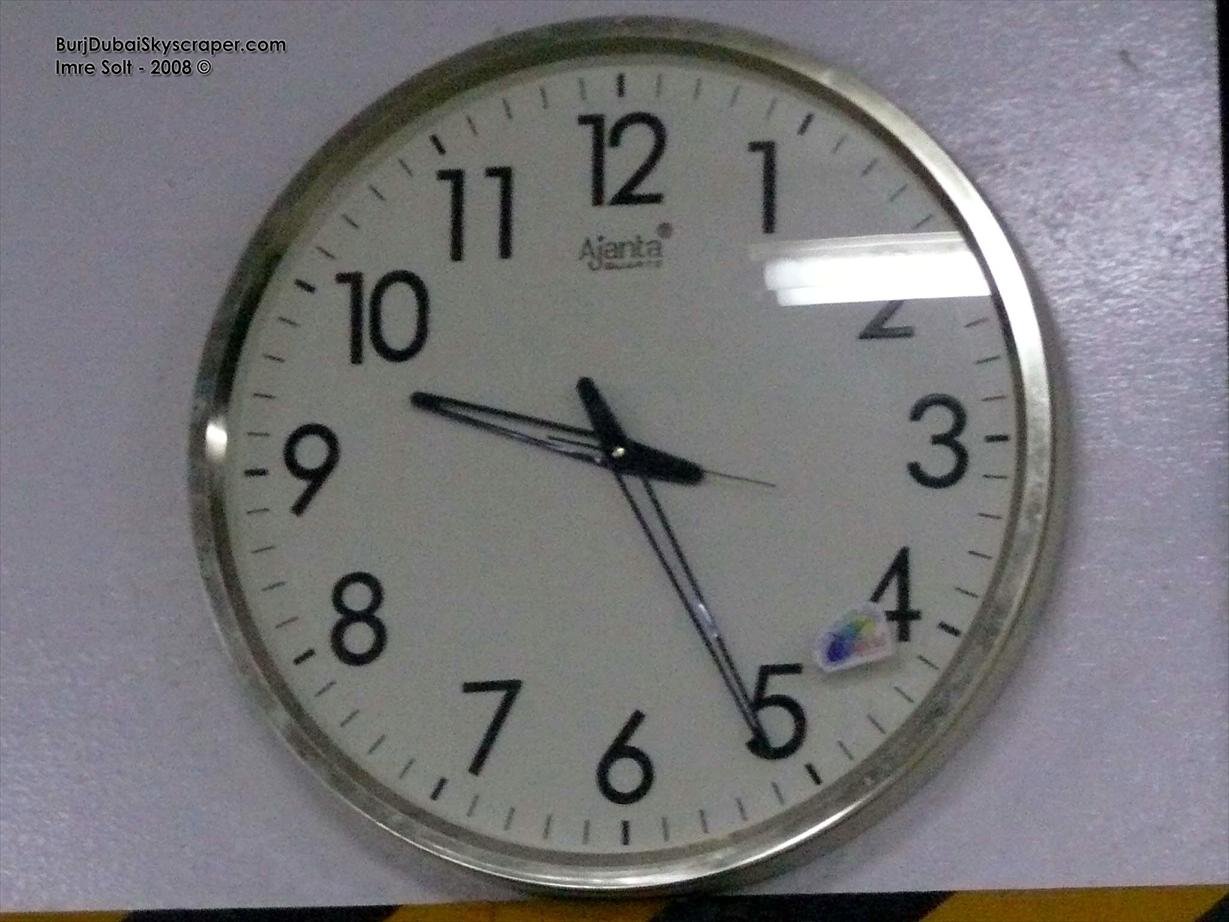The photograph captures a wall-mounted clock that you might typically find in a school or an office; it features a classic design. The clock has a chrome, silver border encircling a white face marked with black numerals (1 to 12). The time is clearly displayed as twenty-five past nine with thin black hands that resemble double strips of metal.

Notably, a sticker is affixed to the glass between the numbers 4 and 5, adorned with mauve, blue, green, and pink colors. However, the specifics of what the sticker depicts are unclear. The clock's manufacturer, "Ajanta," is named prominently in the center.

On the left side of the image, in what appears to be a watermark or an identification mark, the text "Bur Dubai Skyscraper.com, Imre Salt – 2008" is written in black. The clock is mounted on a painted white wall, and at the bottom of the image, black and yellow chevron markings suggest an area designated for caution, possibly indicating a zone where safety is a concern. This setup hints that the location could be at a bus or train station.